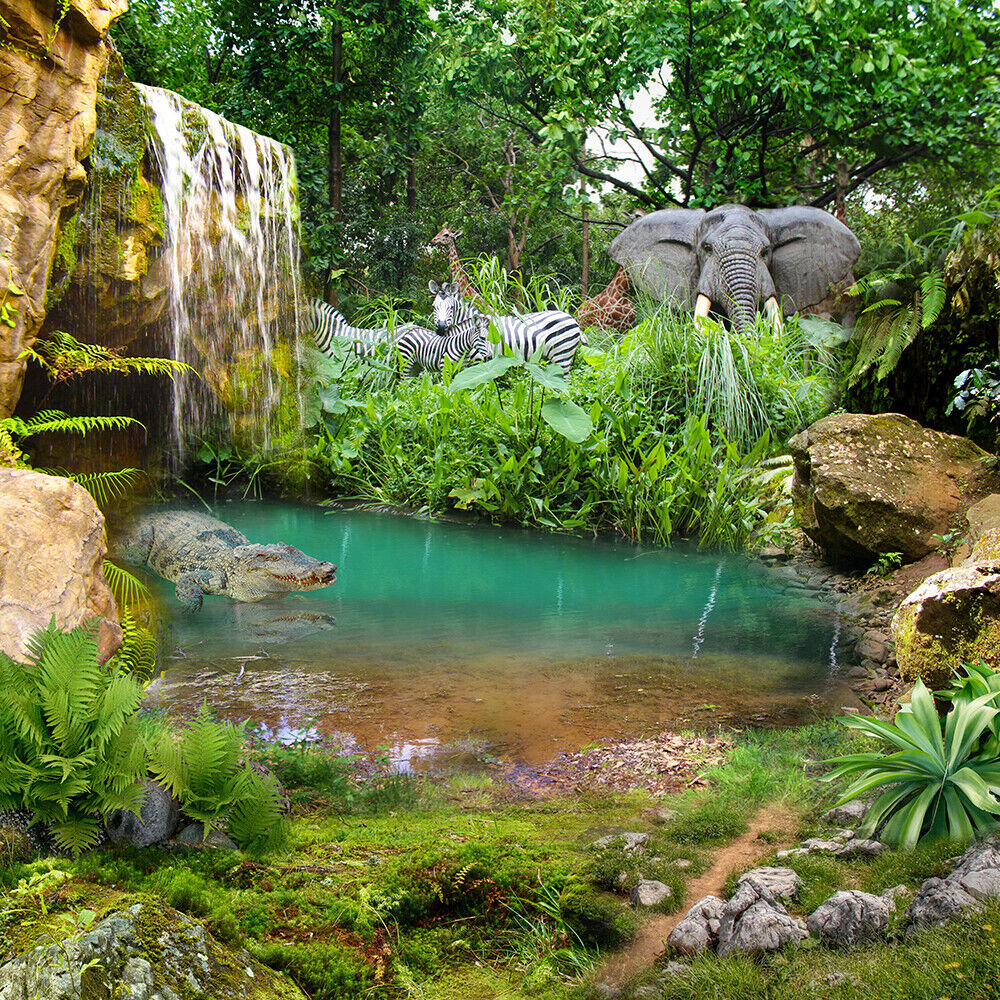The image is a detailed and vibrant depiction of a natural setting, possibly a lagoon in Africa or Asia, teeming with various animals. In the foreground, the scene is rich with lush green plants, grasses, and a variety of rocks—gray and tan—covered in moss. Spanning across the top of the image is a canopy of green trees with brown stems and branches, set against a whitish-gray sky.

On the left side, there is a pond with brown sand visible through the shallow light green water, where an alligator swims, its dark green body barely breaking the surface. Above the alligator, a waterfall cascades over a tan and brown rock formation, with green foliage flanking each side. The water appears white as it tumbles down.

To the right edge of the pond, rocky shores give way to a cluster of flora, intertwining with the habitat of several animals. Strategically placed amidst the greenery is a majestic elephant, partially obscured by thick bushes, with only the upper portion of its head and trunk visible. Nearby, three zebras stand out with their black and white stripes: two facing left and one facing right. Further in the background, almost hidden behind the zebras, two giraffes extend their necks, their heads barely visible above the treetops.

Overall, the scene combines elements of wildlife and natural beauty, portraying an array of animals peacefully coexisting in a seemingly surreal yet captivating landscape.